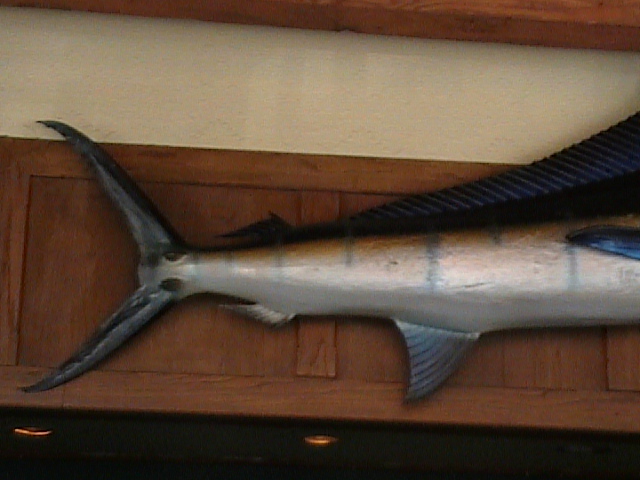The photograph features a taxidermied marlin, prominently displayed on a wall adorned with wooden paneling and white drywall above. Only the tail end of the fish is captured in the frame, starting from the midsection of its body to its sharp, two-pronged tail fins that curve like a backward "C." The marlin's body is primarily a shiny, light gray with distinct vertical blue lines running down its sides. Its robust dorsal fin is a solid dark blue, while two small fins protrude from its belly, adding to the intricate details. The setting appears to be a man cave, living room, or office, with the fish mounted high on the wall near the ceiling, as indicated by the presence of lights below the wooden paneling.